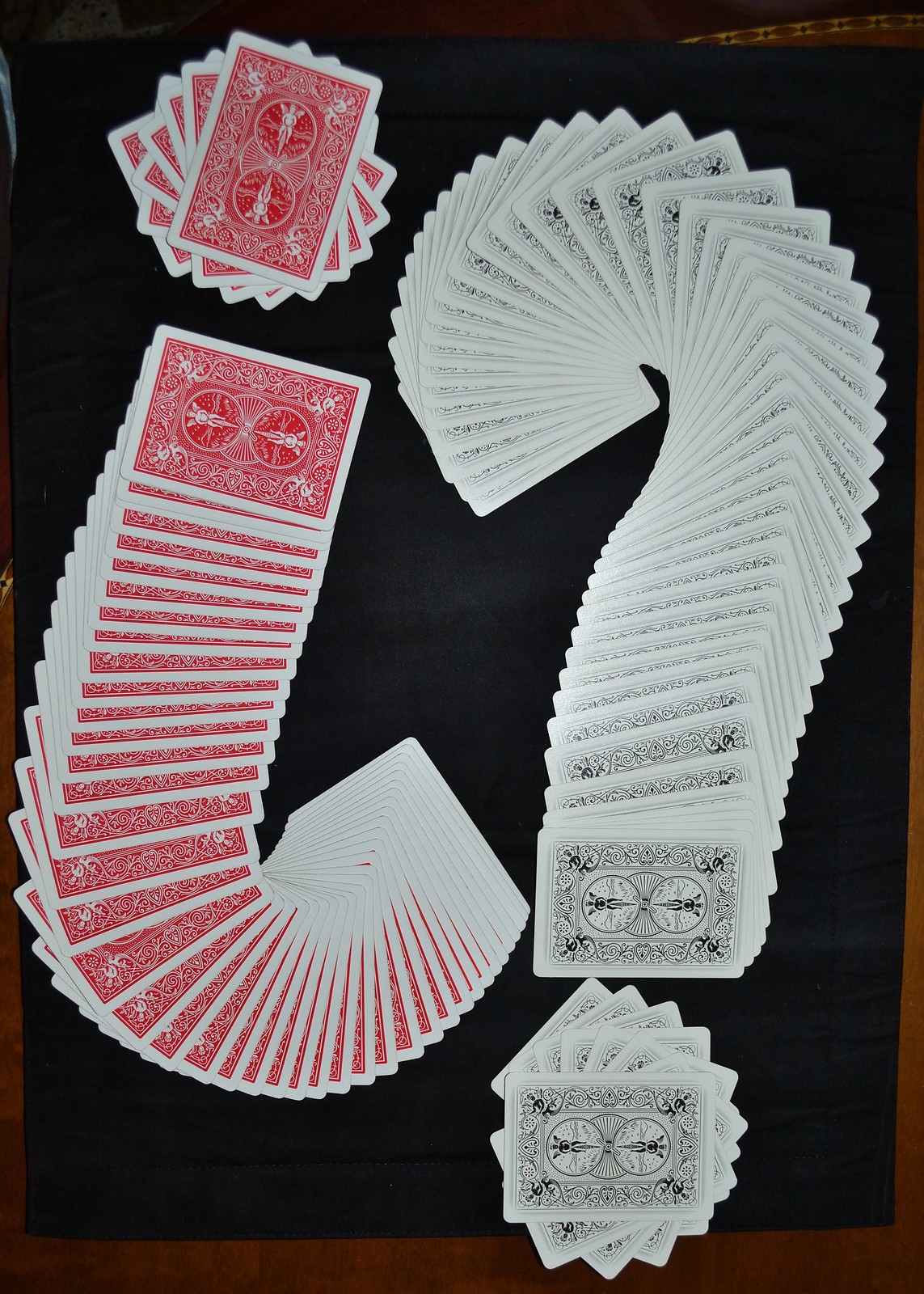In this image, we see two intricately arranged decks of cards displayed on a black dust mat placed on a wooden table. On the left side, the cards have red backs adorned with designs of angels, swirls, and hearts. These cards are meticulously laid out to form an upside-down question mark, with the dot made up of a tightly spiraled group of cards. 

On the right side, another deck features the same elegant designs, but in a monochrome black and white palette. These cards are arranged in the shape of a standard question mark, mirroring the style of the left deck with a spiral dot and a carefully curved body. The arrangement showcases a high level of precision, allowing the cards to flow seamlessly from the top curve down to the line that meets the dot, creating an aesthetically pleasing and organized display.